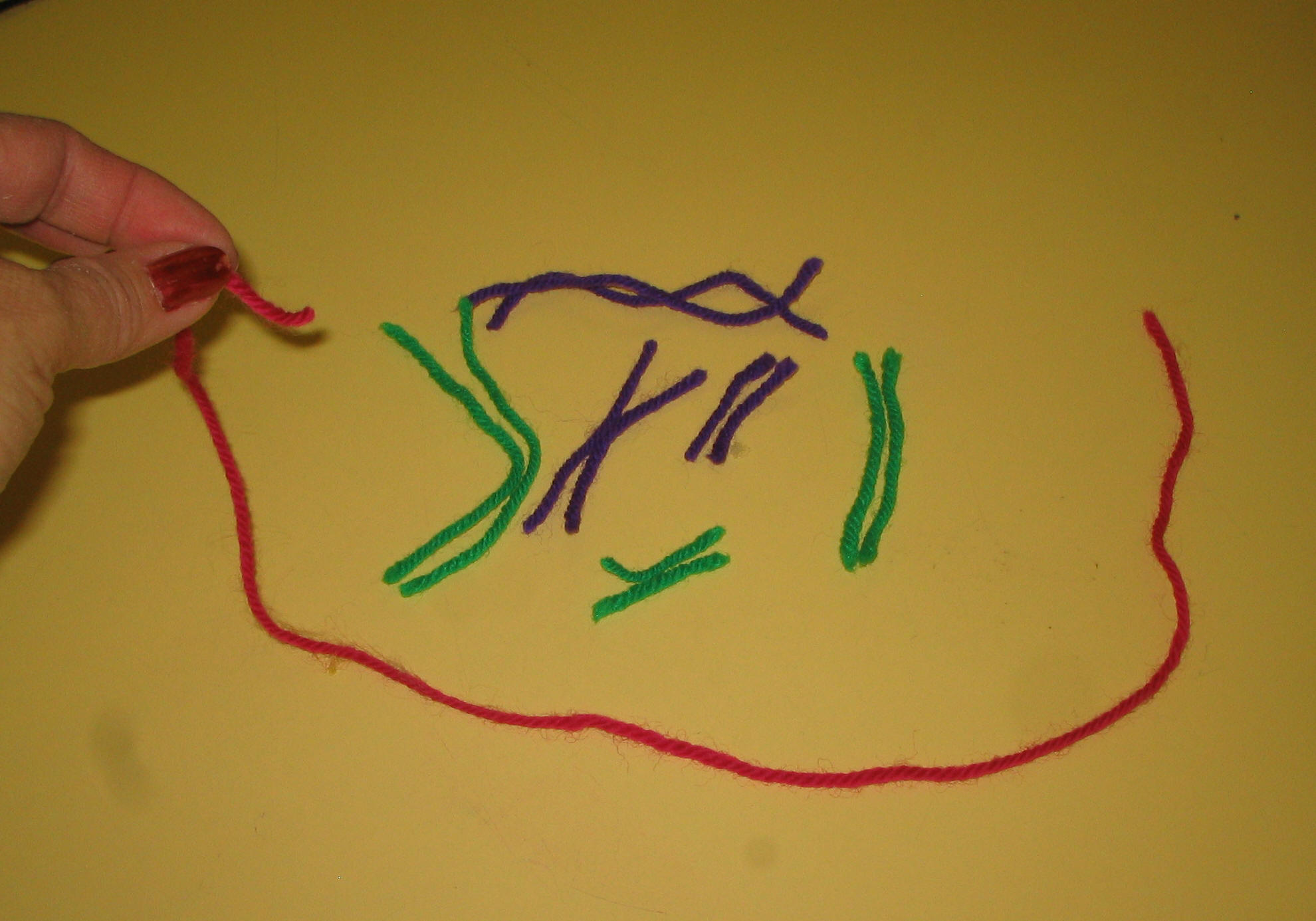The photograph captures a detailed scene of an arts and crafts project involving yarn. A woman's left hand, adorned with chipped red nail polish, is prominently featured on the left side, holding a long piece of red yarn between her index finger and thumb. The background is a yellow or manila-colored surface, possibly a manila folder, which has some visible stains. Surrounding the red yarn in her hand are various short pieces of yarn in purple and green. Specifically, there are two crisscrossed purple pieces at the top, four other pieces of green yarn situated next to these, along with other purple and green yarn snippets scattered around, ranging in length from one to three inches. The arrangement of the yarn pieces somewhat resembles a mouth or a smiley face, indicating a potential design in progress rather than a knitting project.